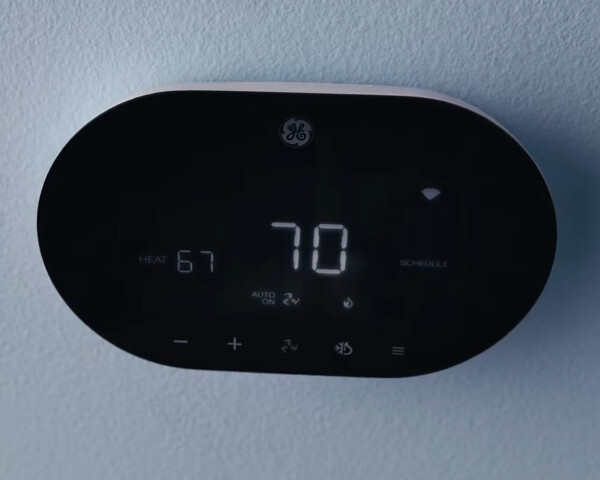A thermostat is mounted on a white textured wall. The device itself is white, blending seamlessly into the wall, but the interface is a sleek, dark black digital display that makes the information stand out vividly. The temperature is set at a comfortable 70 degrees. On the left side of the display, the word "heat" is faintly visible with a current reading of 67 degrees, indicating the heating system's status. On the right side, the word "off" is subtly indicated, along with a triangle icon in the top-right corner, which is not brightly lit and is somewhat hard to distinguish. Below this, there's an icon of a fan with the word "auto" next to it, showing the fan setting. At the bottom of the digital interface, there's a horizontal line featuring several symbols: a minus sign, a plus sign, a fan icon, and a couple of faint emblems that are difficult to see clearly. The plus and minus buttons are likely used to adjust the temperature settings.